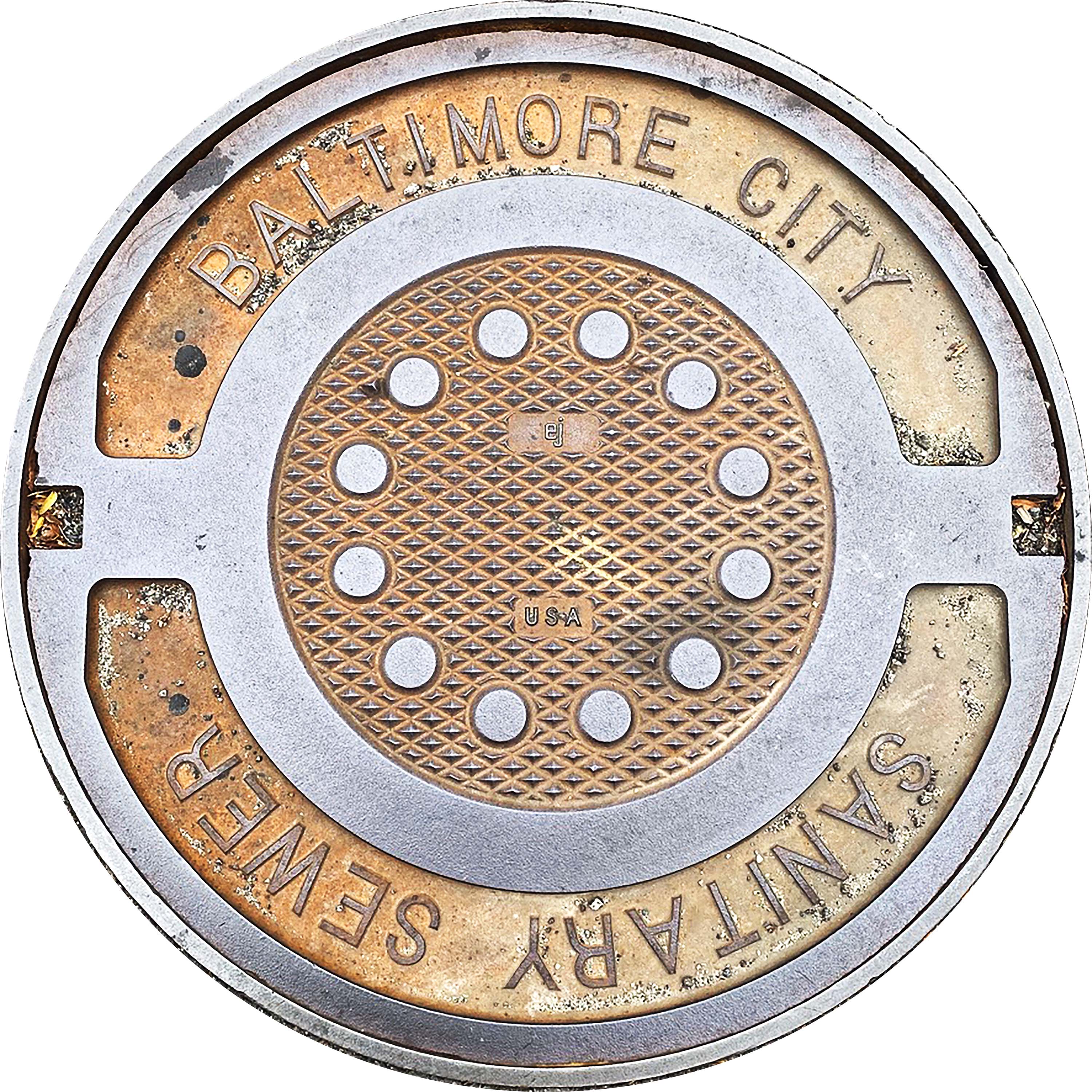The image features a weathered, round steel manhole cover, typically found on city streets, designed to withstand foot and vehicle traffic. The cover belongs to Baltimore City, as indicated by the words "Baltimore City" emblazoned on the top part of the steel plate and "Sanitary Sewer" marked on the bottom. The cover shows clear signs of aging and long-term use, with noticeable rust, dirt, and grime. Gravel and small rocks have lodged into various crevices, particularly around the raised diamond patterns and notable bronze areas. In the center of the cover, there is a distinctive circular design with the word "USA" inscribed. Two notches on either side hint at the tools needed to lift the cover for sewer access. Set against a stark white background, the photograph isolates the manhole cover, highlighting its simplicity and utilitarian wear.